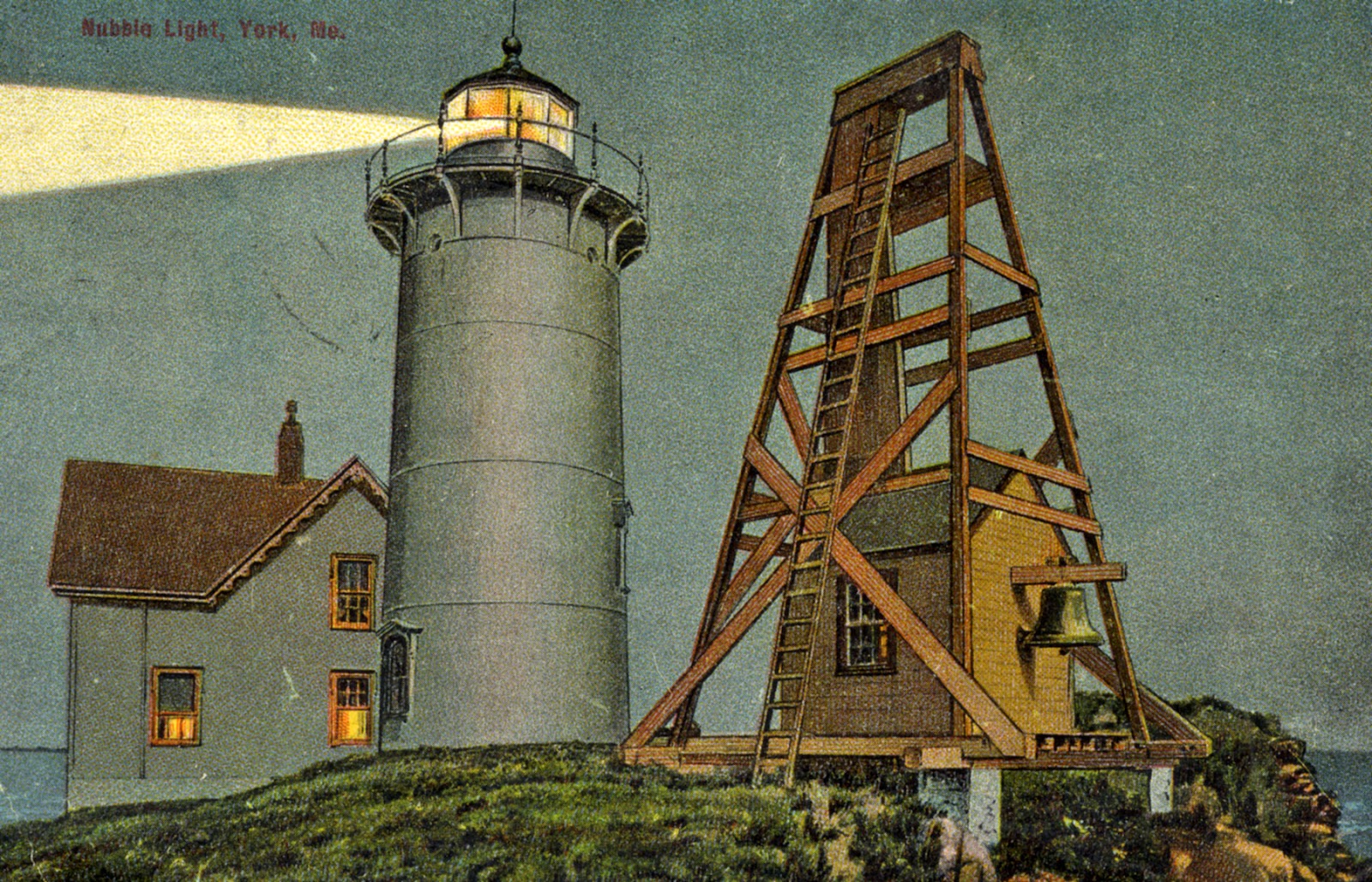The image showcases a historic, faded watercolor painting of a lighthouse situated on a small knoll above the ocean. The lighthouse, a thick structure painted in a gray color, features a black balcony near the top and a glass section emitting an orange-yellow light streaming to the left. The painting is titled "Nubby Light, York, Maine" as indicated in the top left corner, with Maine abbreviated as M-E.

Adjacent to the lighthouse, there's an A-frame structure with a tall brown ladder leading to the top, significant for its substantial size and featuring a large gold-colored bell on its side. Below the A-frame, a small shack can be seen. To the rear of the lighthouse, a two-story house painted in the same gray color is present. This house has a distinctive brown roof, three windows with lights on in the bottom two, and appears to add depth to the maritime scene. The overall depiction suggests an aged, historic atmosphere with dark, subdued colors capturing a serene coastal environment.